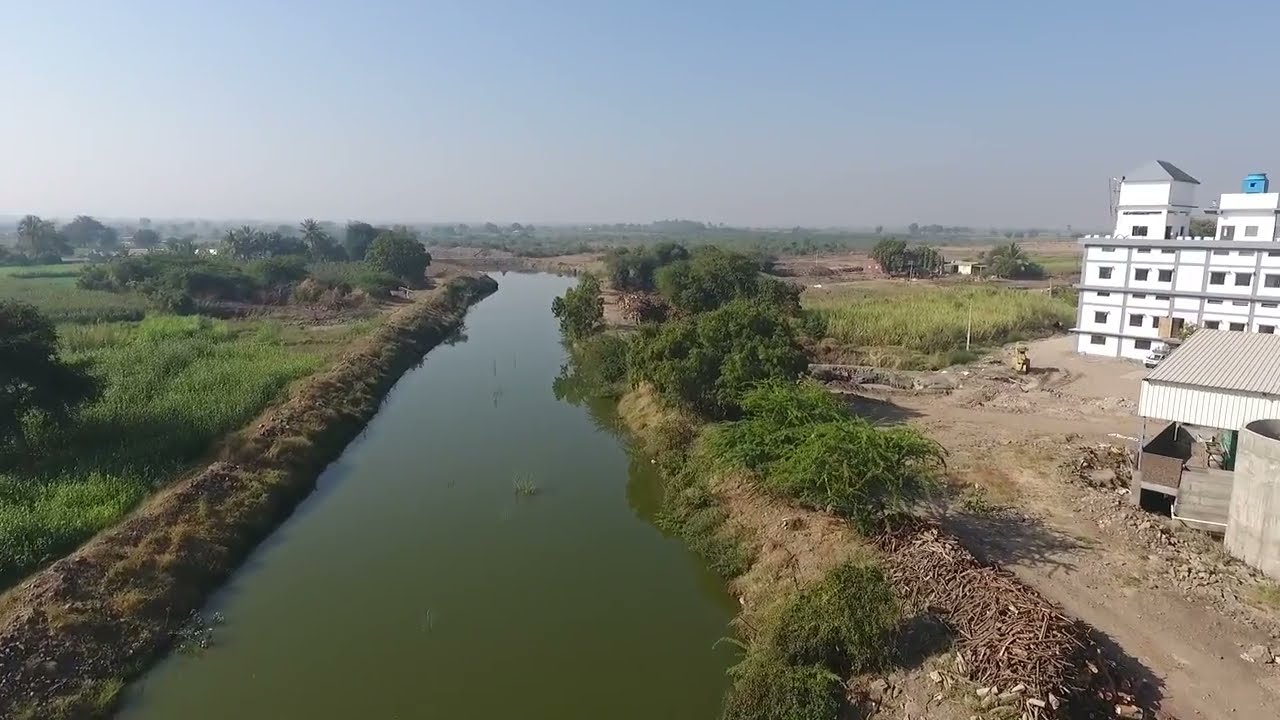The photograph presents a serene, outdoor scene on a slightly hazy day. Central to the image is a wide, murky stream or canal with stagnant, brownish-green water. The left bank is a raised, brown dirt mound leading up to a patch of taller green grass and a grassy field, lined with occasional trees. On the right bank, there is a dirt path or road wrapping around the area. Adjacent to this path is a tall, white building, approximately four stories high, potentially an apartment or industrial building, with a large gray-roofed shed or metal structure in front of it. This metal structure consists of a few support beams and a roof. Farther right, there is a cylindrical silo, adding to the industrial feel of the setting. The backdrop features more trees and a clear, blue sky, contributing to the calm ambiance of the scene. The picture lacks any people or text, focusing solely on the natural and built environment.